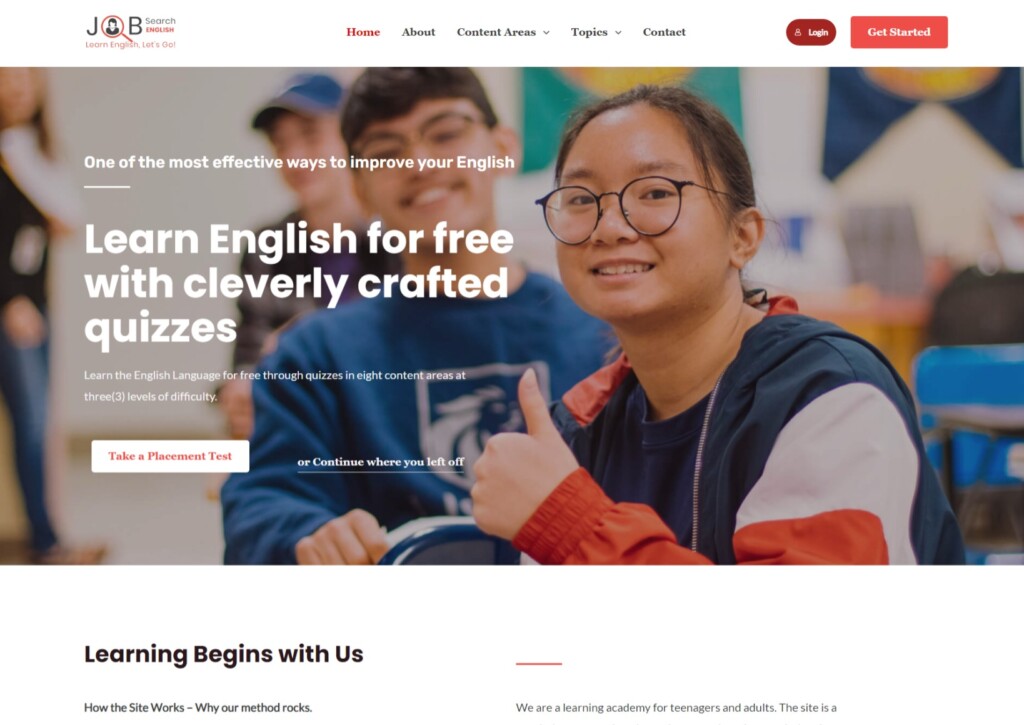"JB Cedric English: Learn English - Let's Go!

At the top of the page, a sleek white navigation bar features various options. The 'Home' section is highlighted in red, while the other sections - 'About,' 'Content Areas,' 'Topics,' and 'Contact' - are listed in black to the right. Beside this, there is a burgundy login button and a prominent red 'Get Started' rectangle.

Below the navigation bar, images showcase students in a vibrant classroom filled with colorful flags adorning the back wall. The students appear enthusiastic and engaged, embodying the tagline, 'One of the most effective ways to improve your English.'

In large, bold white lettering overlaid on the left side of the image, the text reads, 'Learn English for free with cleverly crafted quizzes.' Further details highlight that users can learn English through quizzes in eight content areas, with three levels of difficulty.

A white tab on the left with red lettering invites users to 'Take a Placement Test,' while a clickable option to 'Continue where you left off' is to the right.

A happy student with a thumbs up signals approval below the heading 'Learning begins with us,' emphasizing the site's focus on effective learning methods. Additional sections explain 'How the Site Works,' 'Why Our Method Rocks,' and offer opportunities to 'Learn More About Us,' reinforcing that the platform is a dynamic learning academy for both teenagers and adults."